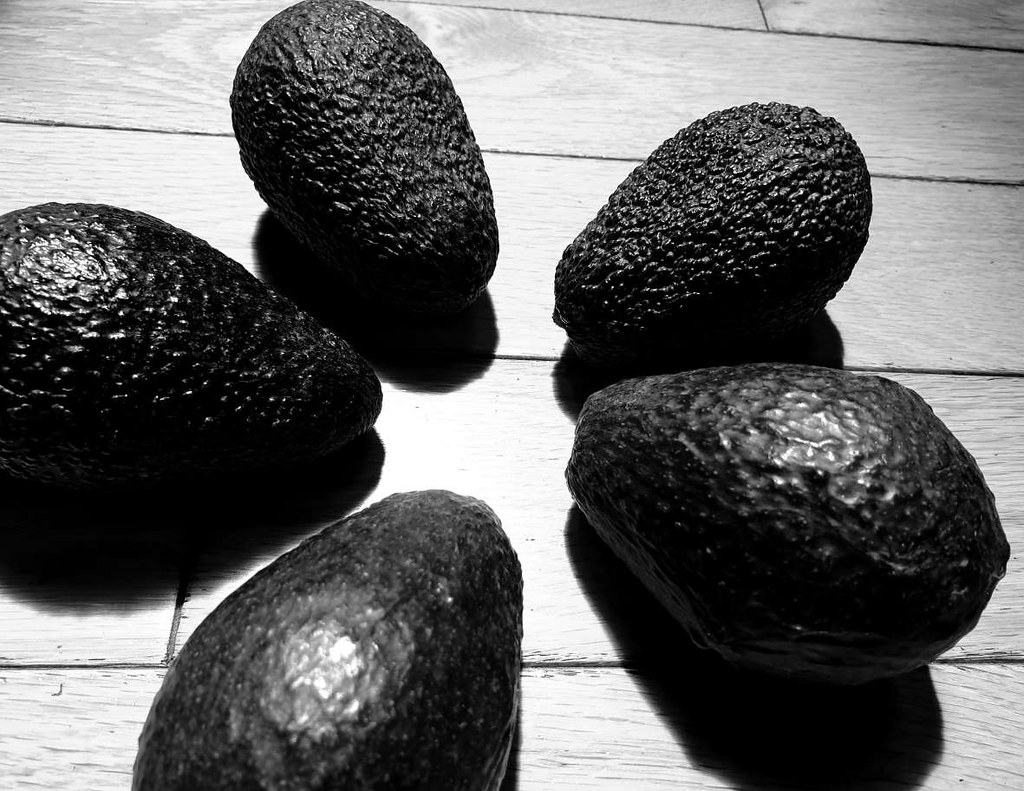In this black and white photograph, five avocados are artfully arranged in a circular, flower petal-like pattern on a wooden floor. The hardwood floor's detailed grain is clearly visible, with each plank and connecting line discernible beneath the avocados. The avocados toward the bottom of the image appear smooth, with light accentuating their sleek textures, while those at the top display rougher, more wrinkled surfaces, enhanced by the interplay of light and shadow. The avocados are uncut, with their pointy tips converging at the center, forming a star-like arrangement. Despite the monochrome palette, which renders the avocados dark, possibly black, the intricate textures and shapes are captured with striking clarity.